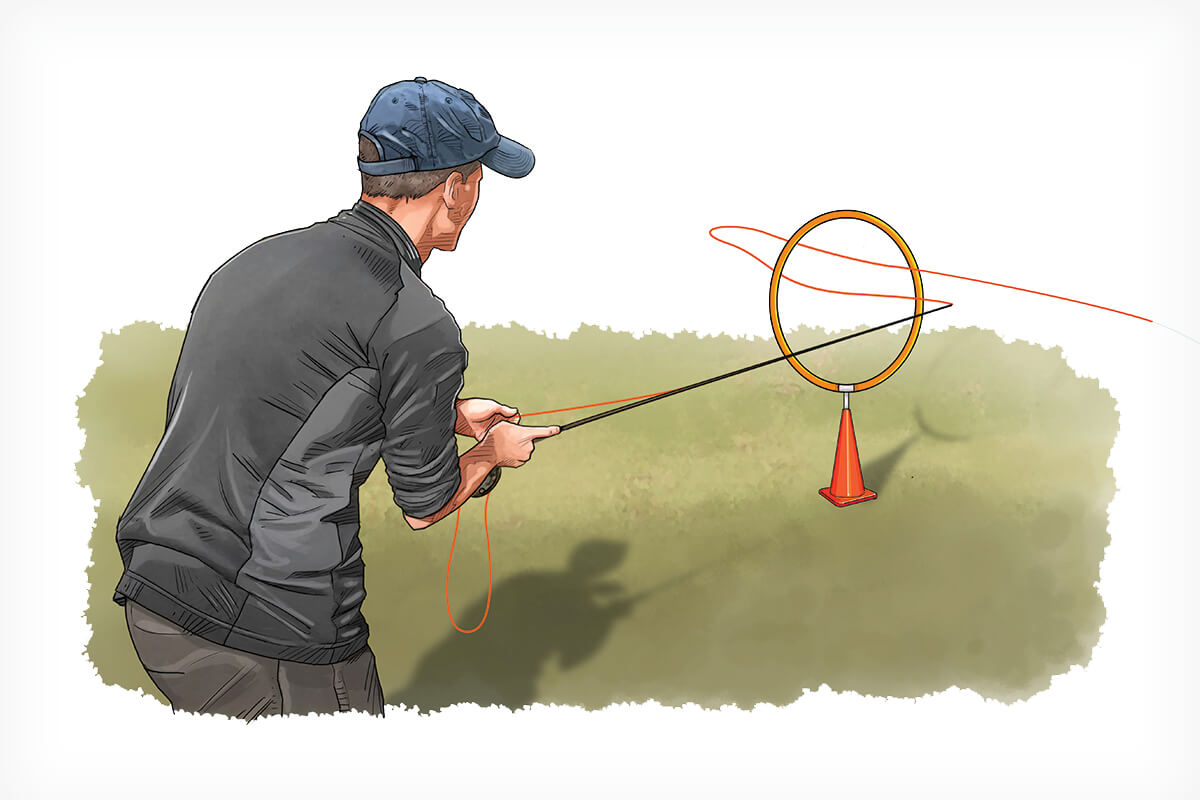In this animated, cartoon-like artwork set against a white backdrop, a man stands on a grassy area, depicted from behind. He is wearing a blue cap, a dark gray to light black shirt, and brown pants that are cropped at the bottom edge of the image. The man holds a fly casting rod in his right hand, while his left hand grasps the fishing line. In front of him is an orange caution cone with a light orange hoop mounted on top. The fishing line zigzags through the hoop, extending out and curving back to the right side of the image, transforming into a light gray hue before disappearing off the canvas. His shadow on the ground indicates that the sun is behind him, adding depth to the scene where he practices casting his line in an attempt to thread it through the hoop.